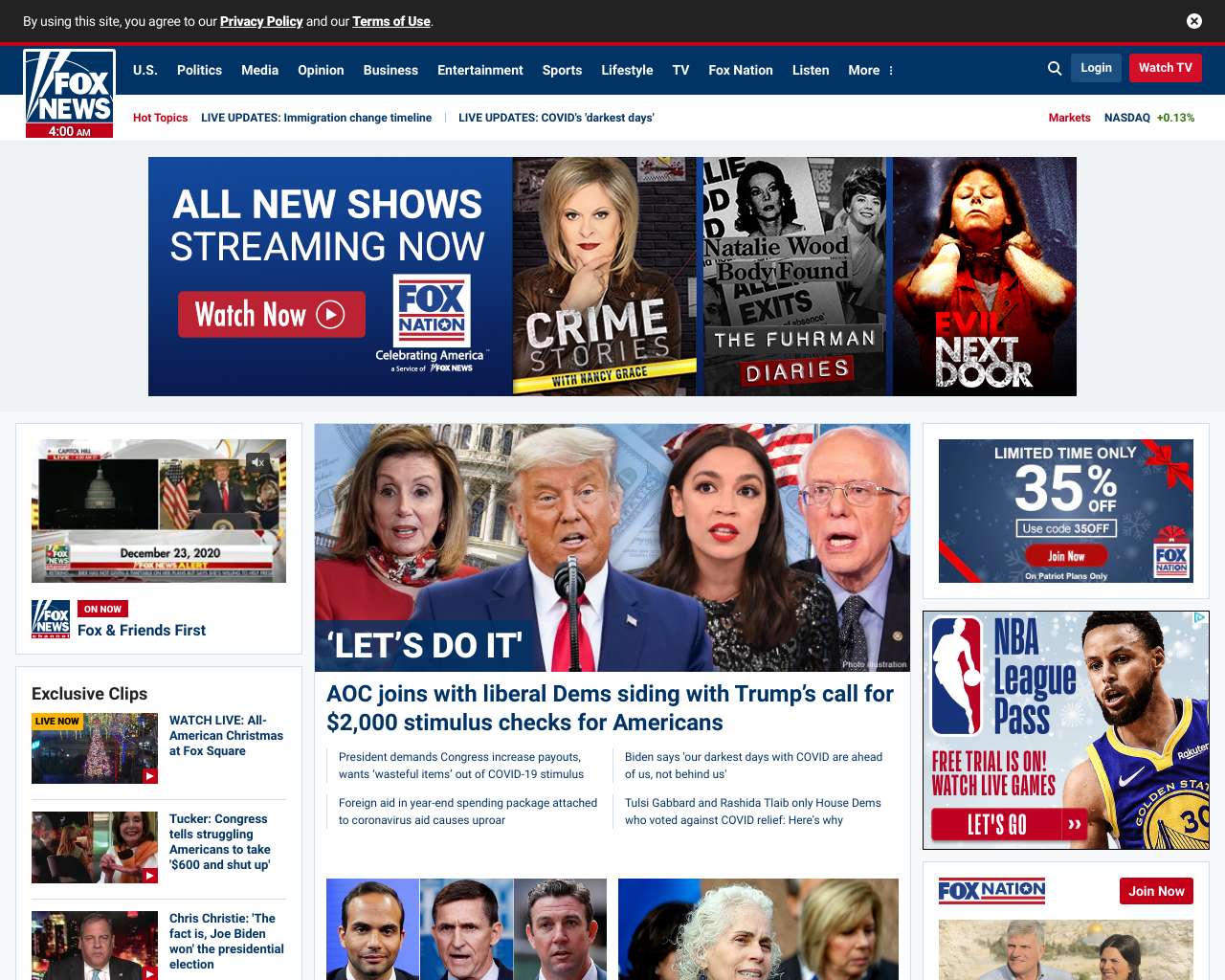This is a detailed look at the Fox News website as displayed early in the morning at 4 AM. At the top of the site, a banner informs users that by using the site, they agree to the privacy policy and terms of use. Prominently displayed is the Fox News logo. Below this banner is a blue navigation bar with various categories such as US Politics, Media, Opinions, Business, Entertainment, Sports, Lifestyle, TV, Fox Nation, Listen, and more. Users are also given the options to log in and watch TV.

One of the key promotions on the site reads "All New Shows Streaming Now" with a "Watch Now" button leading to Fox Nation's special features including titles like "Celebrating America," "Crime Stories with Nancy Grace," "The Furman Diaries," and "The Evil Next Door." 

Beneath these promotions is a timestamp marked December 23rd, 2020. Featured prominently are two images: one of the White House and another showing former President Donald Trump speaking behind a podium. Adjacent to these images are smaller photos of Bernie Sanders, Alexandria Ocasio-Cortez (AOC), Trump, and Nancy Pelosi.

An attention-grabbing headline reads "Let's Do It - AOC Joins with Liberal Dems Siding With Trump's Call for $2,000 Stimulus Checks for Americans." Additionally, a promotion at the bottom of the page offers a free trial for the NBA League Pass.

This comprehensive layout provides a snapshot of the key features, offerings, and current news highlighted by Fox News early on this specific date.